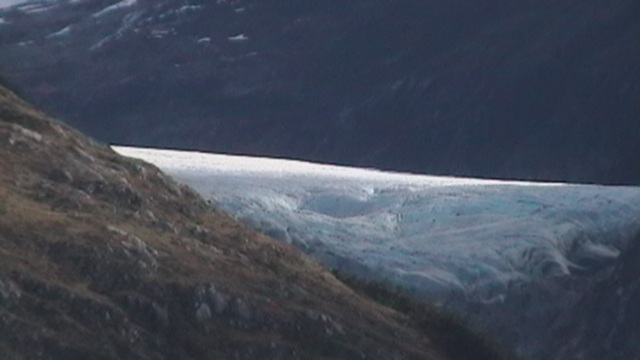The image depicts a rugged landscape, with a dramatic contrast between various geological features under natural lighting. In the foreground, occupying the lower left portion, there is a rocky hillside or cliff that is brown and speckled with gray rocks and patches of grass, though the coloration appears somewhat dark and almost black in parts. This hillside is crisscrossed with bridges, adding a man-made touch to the natural scenery.

Dominating the middle of the image is a glacier that stretches down a valley between two large, dark mountains. The glacier's surface is white and jagged, evoking the appearance of a frozen waterfall cascading through the landscape. The glacier is prominently positioned in contrast to the darker, rocky mountainous region in the background, which appears almost black with patches of shadow cast by the surrounding cliffs.

The overall scene is captured on a bright day, though shadows from the tall cliffs partially obscure the glacier, emphasizing the stark lines and natural ruggedness of the terrain. The different layers of color—browns, grays, whites, and some blues—blend to present a vivid tableau of a cold, dramatic outdoor scene.